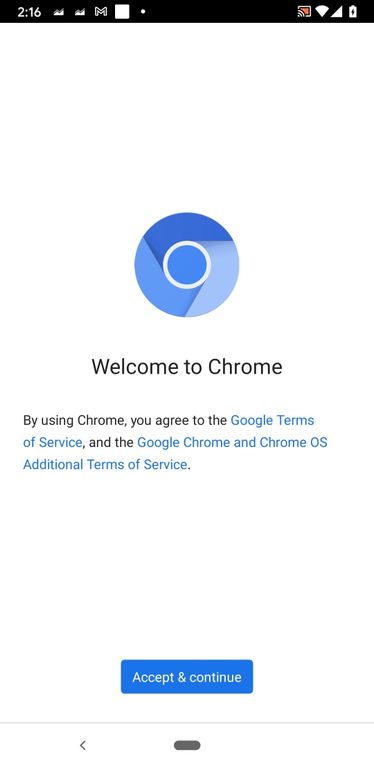The image displays a screenshot taken from a cell phone. At the top, within a black rectangle, the time "2:16" is prominently visible, positioned on the left side alongside a few additional icons. To the right, the battery indicator shows that the phone may need charging. 

In the central area of the screen, there's a welcome message for the Chrome browser. The typically colorful Chrome logo is replaced with a unique monochromatic design: a central periwinkle circle encircled by a white ring. A darker periwinkle hue is located at the top of the circle, gradually fading to a lighter shade around its circumference.

Below the logo, in black text, it reads "Welcome to Chrome". Further down the screen, also in black text, it states: "By using Chrome, you agree to the Google Terms of Service and the Google Chrome and Chrome OS additional terms of service."

At the bottom of the image, there is a blue button with white text stating "Accept and Continue".